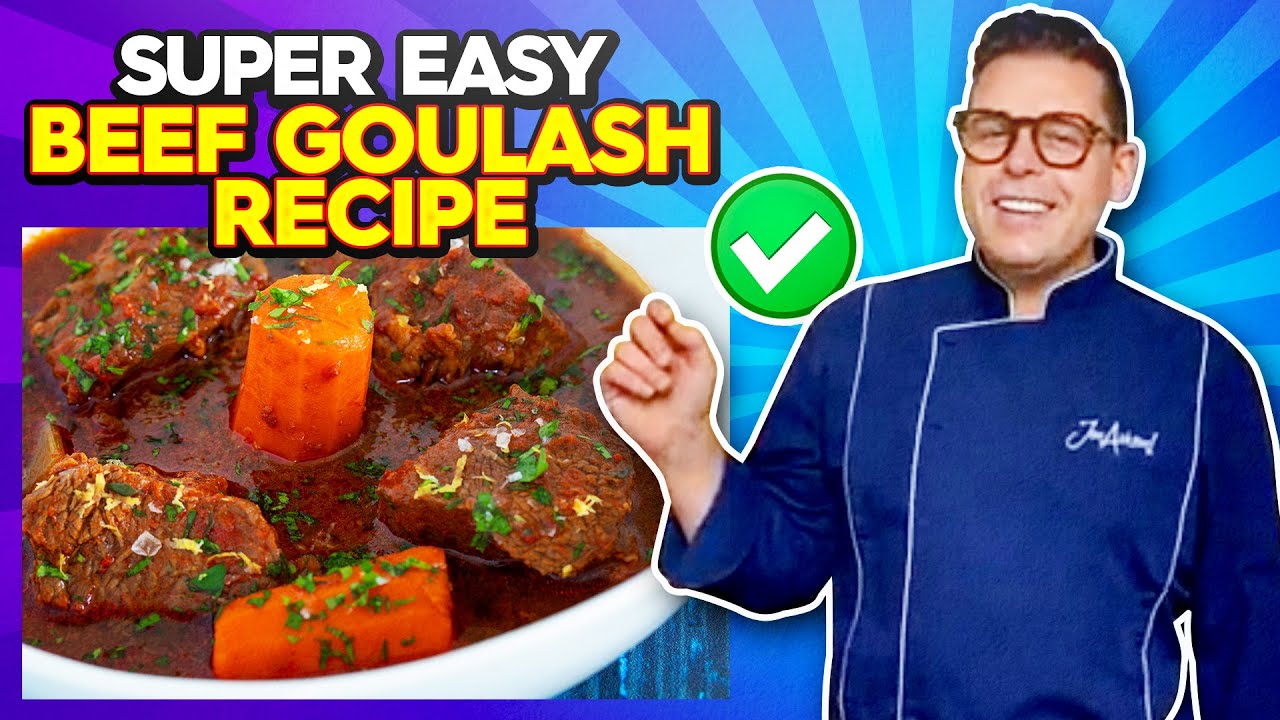The image is a colorful advertisement featuring a vibrant background with blue and purple alternating stripes, reminiscent of a pinwheel. On the left side is a white ceramic bowl filled with a hearty beef goulash, featuring chunks of brown beef and two slices of carrot, one upright and one laying down, adorned with greenery and lemon zest. Above the bowl, bold white capital letters declare "SUPER EASY" against a shadowed backdrop, and below in yellow letters with red and black borders, it reads "BEEF GOULASH RECIPE." Centered between the bowl and a man is a green circle with a white check mark. To the right, a smiling mid-30s man with short brunette hair and maroon glasses wears a blue chef's jacket with white piping and an apron. His right hand is slightly raised and bent at the elbow, fingers curled inward. The overall layout suggests it's a clickable online banner or YouTube cover for an easy beef goulash recipe.